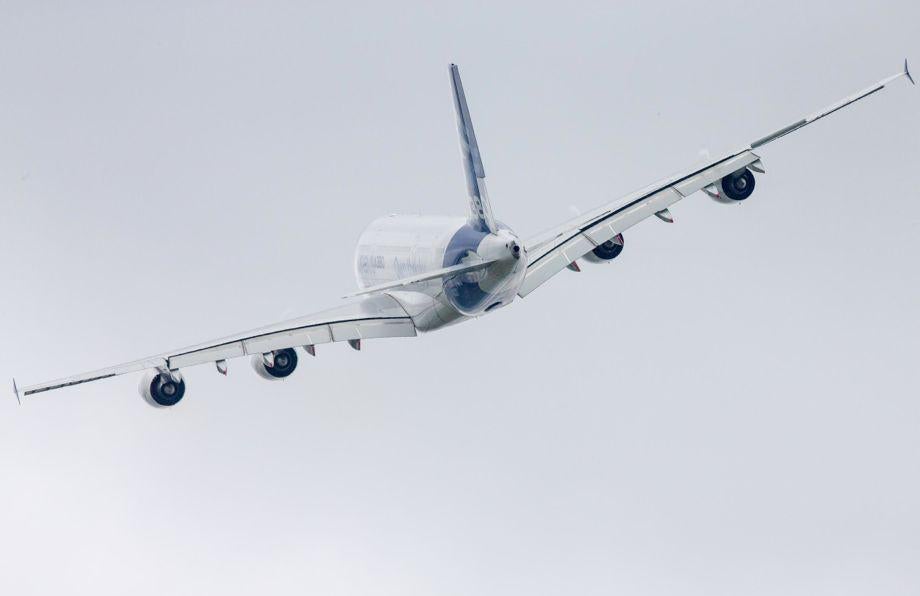The image depicts a small airplane mid-flight against a light gray, cloudy sky. The airplane is predominantly white with accents of bluish-gray and features a large blue fin on the tail. Each wing, slightly tilted to the left, houses two black engines. The wings and fuselage are also tinged with hints of gray. The plane appears to be either ascending or descending, though its precise motion is unclear. There is no visible writing or markings on the airplane, which occupies the majority of the frame.